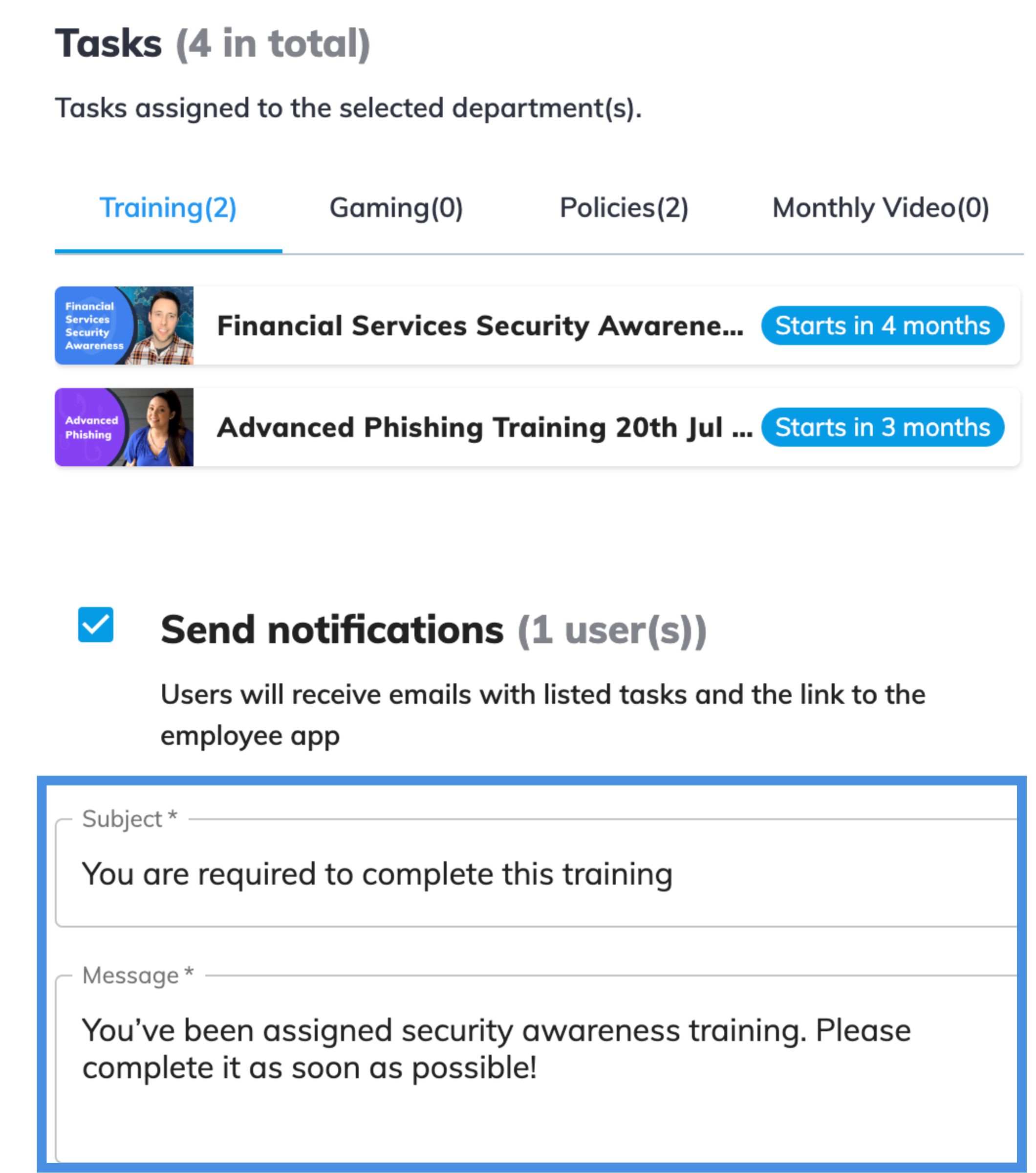The image is a screenshot of a web page with a white background. In the top left corner, the word "Tasks" is written in black font, followed by "4 in total" in gray font within parentheses. Below this, in gray font, the text reads "Tasks assigned to selected departments."

Below this heading, there is a horizontal menu featuring four items: 
1. "Training (2)" in blue font
2. "Gaming" in gray font
3. "Policies (2)" in gray font
4. "Monthly Video (0)" in gray font

Further down, in bold black font, the text "Financial Services Security Awareness" is partly visible, with some letters of "Awareness" cut off. Following this, there are two items listed:
1. "Advanced Phishing Training" - Dated "20th JUL" (20th of July)
   - To the right, a blue rectangle with rounded edges contains the text "Starts in 4 months" in white font.
   - On the left, a small photo presumably of the instructor: a white man in a plaid shirt.
2. "Another Task" - (Details not fully provided)
   - To the right, a blue rectangle with rounded edges contains the text "Starts in 3 months" in white font.
   - On the left, a photo of a white woman with dark brown hair wearing a blue shirt.

Below this section, bold headlines read "Send Notifications." To the left, there is a blue box with a white check mark and the text "Users will receive emails with listed tasks and the link to employee app." This content is enclosed within a blue rectangle line.

The next section includes fields for "Subject" and "Message."
- Subject: "You are required to complete this training."
- Message: "You've been assigned security awareness training, please complete it as soon as possible."